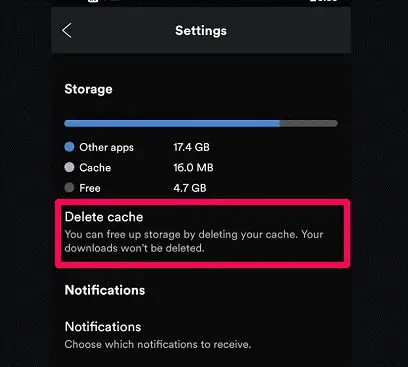This image captures the settings screen of the Spotify mobile app, specifically within the storage management section. The interface features a black background with white text, maintaining a clean and readable aesthetic. At the top of the screen, there's an option labeled "Delete Cache," accompanied by an explanatory note indicating that this action will free up storage space by removing cached data without affecting any downloaded content.

The cache currently occupies a mere 16 megabytes of storage. Beneath this, a visual storage bar illustrates the distribution of storage usage: a dominant blue section represents "Other Apps" consuming a substantial 17.4 gigabytes, a green segment indicates 4.7 gigabytes of free space, and a tiny sliver at the very end signifies the relatively negligible space taken up by the Spotify cache.

As you scroll further down, additional settings options appear, such as "Notifications," where users can customize which notifications they wish to receive. A back button is also present for easy navigation. This detailed interface helps users manage their device’s storage efficiently while using the Spotify app.